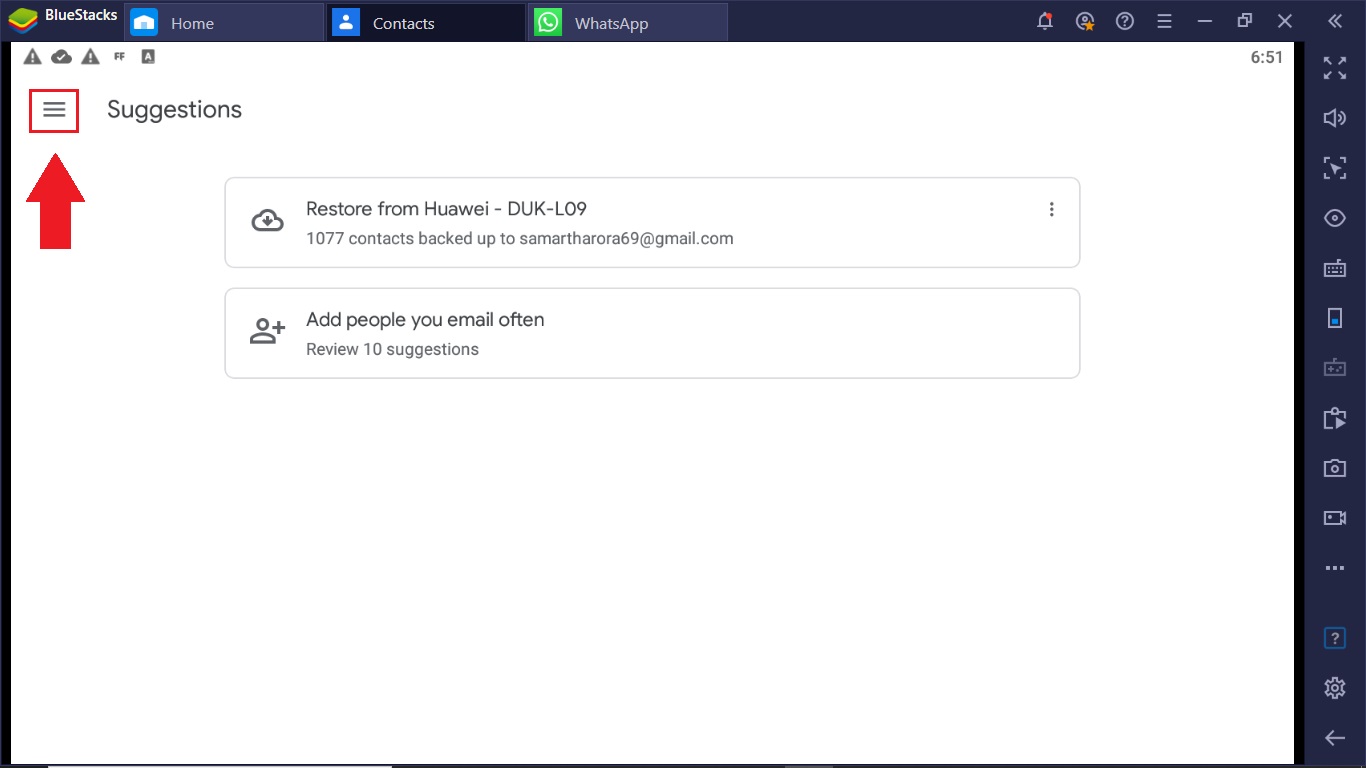The image showcases the BlueStacks interface. In the top left corner, the BlueStacks logo is prominently displayed, featuring colorful blocks stacked in a pattern with green, yellow, red, and blue hues. To the right of the logo, there are several icons with corresponding labels: a blue icon with a house labeled "Home," a blue box with a white person icon labeled "Contacts," and a green box with a speech bubble and white phone icon labeled "WhatsApp."

In the top right corner, there are multiple icons including a bell with a red notification dot, a question mark within a circle, three horizontal lines, two small boxes, an "X," and a couple of arrows. Along the right side of the interface, other icons are vertically arranged: arrow pointers in various directions, a speaker symbol, an eyeball icon, a keyboard icon, a camera icon, a gear, and an arrow pointing to the left.

On the left, within a large white area, three horizontal lines are situated in the top left corner and encased in a red border with a red arrow pointing towards them. Next to these lines, the word "Suggestions" is displayed. Below this, there are two boxes: the first one states "Restore from Huawei DUK-L09 1,077 backups or contacts backed up to samartharora69@gmail.com," and the second box reads "Add people you email often, review 10 suggestions."